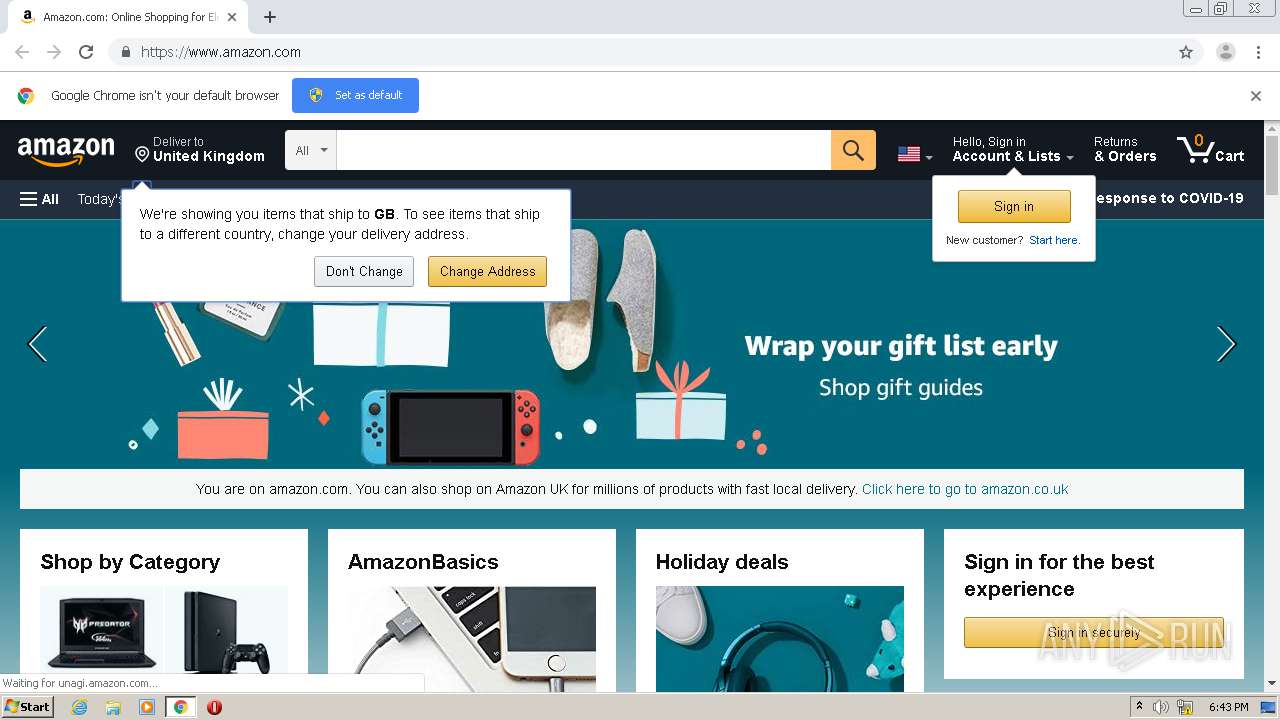This image captures a detailed view of the Amazon.com web page as seen through the Chrome browser.

At the very top, the browser tab reads "Amazon.com: Online Shopping." Below the tab, the address bar displays "https://www.amazon.com." A notification bar beneath the address bar informs the user that "Google Chrome isn't your default browser," with a blue button labeled "Set as default" on the left and a close (X) button on the right.

The main Amazon page features a black background header. The Amazon logo is positioned to the left, followed by the text "Delivered to United Kingdom." Centered below the header is a prominent, white search bar. To the right of the search bar, a United States flag icon is displayed, followed by the "Hello, Sign in" option, which expands to "Account & Lists" on hover. Next to it, there are "Returns & Orders," and finally, a shopping cart icon with zero items.

Immediately beneath this header is a dialog box stating, "We're showing you items that ship to GB. To see items that ship to a different country, change your delivery address," offering two choices: "Don't change" and "Change address."

Further down, an image carousel promotes various items, including gaming consoles and slippers, under the banner "Wrap your gift list early. Shop gift guides."

A white navigation bar beneath the carousel alerts users: "You are on Amazon.com. You can also shop on Amazon UK for millions of products with fast local delivery. Click here to go to Amazon.co.uk."

The page continues with several categories for exploration, including "Shop by Category," "Amazon Basics," "Holiday Deals," and a prompt to "Sign in for the best experience."